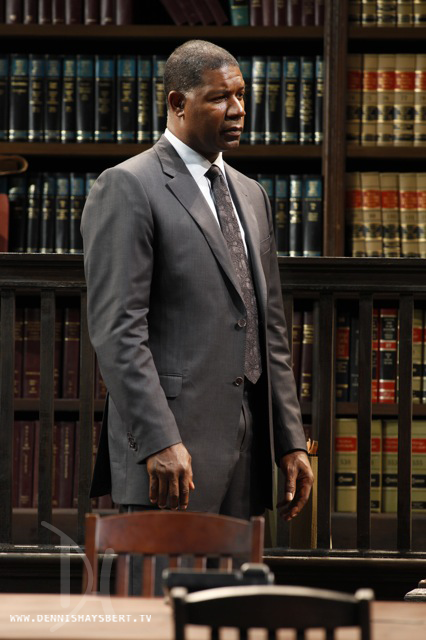In the image, renowned actor Denzel Washington is standing in front of an elegant mahogany bookshelf lined with an array of law books in various colors and sizes. He has short black hair and is dressed impeccably in a gray suit with a white shirt and a gray tie adorned with bronze-ish designs. Behind him, the law books are meticulously organized: the top shelves on the left display dark blue and light blue volumes, while the top shelves on the right feature tan books with orange and blue stripes adorned with gold trims. The bottom shelves on the left hold dark brown and gold books, and those on the right contain black, silver, and gold volumes, with some sporting orange accents. In front of Denzel, there is a sturdy wooden table surrounded by matching chairs. Centrally placed on the table is a landline telephone. A watermark with the text "www.denismaisbert.tv" can be seen in the bottom left corner of the image. Denzel appears to be in a lawyer's office, looking off to the right, exuding a composed and thoughtful demeanor.